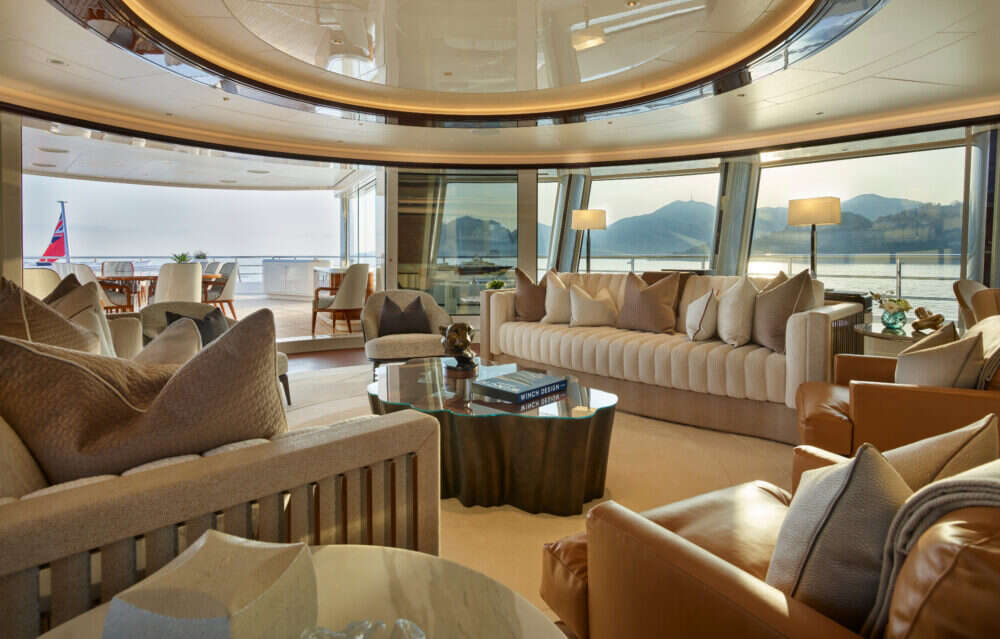This image captures a luxurious lounge area on the deck of a mega yacht, offering a breathtaking view of the open sea through expansive, angled glass windows. The ceiling features a strikingly elegant design with a shiny white circular dome bordered with gold that adds to the opulence of the space. The room is furnished with an assortment of plush seating, including beige sofas adorned with a mix of white and brown throw pillows, a brown leather chair with a gray pillow, and chic upholstered love seats. A large piece of driftwood serves as a unique base for a glass coffee table, which holds a small, intriguing statue of a man holding a globe, along with a coffee table book and other decorative items. The indoor seating area seamlessly transitions to an outdoor deck featuring patio-style dining furniture, perfect for dining with a view of the distant islands and mountain range. The room is further embellished with elegant lamps on each side of the couches, ensuring a cozy and inviting atmosphere for relaxation or reading.